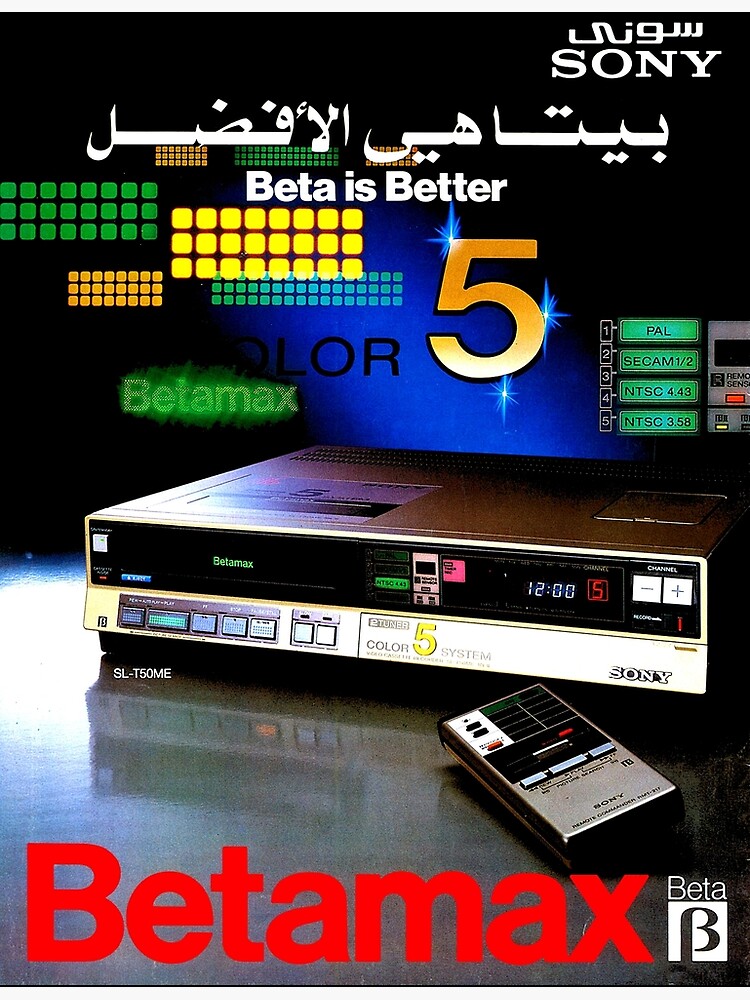This advertisement features an older Sony Betamax video cassette recorder (VCR). The top of the ad showcases foreign text, likely Arabic, followed by the word "Sony." Below this, more Arabic characters are displayed, and then the phrase "Beta is better" appears in English. Prominently, there is a large, shiny gold number "5". Beneath this, the Betamax unit itself is depicted. This rectangular VCR has a silver exterior, marked with "Sony" and "color 5 systems." A flat strip of silver buttons runs along the front, with a black area above likely for inserting the cassette. Features include plus and minus channel buttons on the right-hand side and a built-in clock showing "12:00." Additional text indicates multiple video formats: "1 PAL, 2 CCAM 1.5, 3 and 4 NTSC 4.43, 5 NTSC 3.58." The model number "SL-T50ME" is visible beneath the unit. Accompanying the VCR is a silver and black remote control. At the bottom of the advertisement, in large red font, the word "Betamax" is prominently displayed, along with a small blue and white box containing the word "Beta."